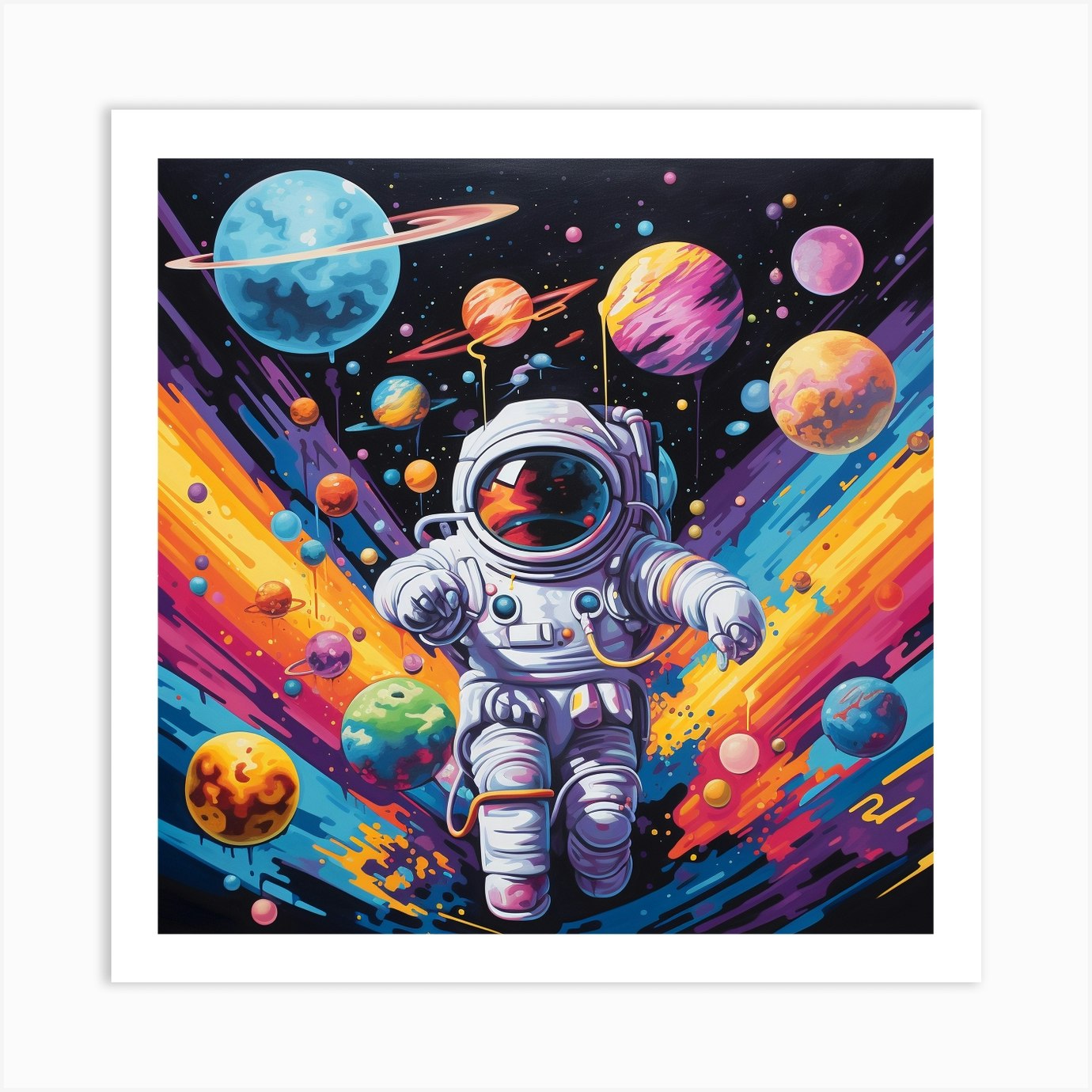This vibrant digital artwork features a cartoon astronaut, clad in a gray spacesuit with a glass helmet and blue circles on the front connected by tubes to a backpack, floating through a whimsical, colorful interpretation of space. Bursts of paint in hues of purple, blue, yellow, orange, and pink form a V-shape around the astronaut, contrasting brilliantly against the dark black sky behind him. The scene is dotted with variously colored planets, stars, and smaller celestial bodies, including a distinctly green and blue Earth. This playful, comic-book-style image evokes a sense of fun and wonder, reminiscent of 1980s animated adventures, and is designed to excite the senses rather than adhere to scientific accuracy.